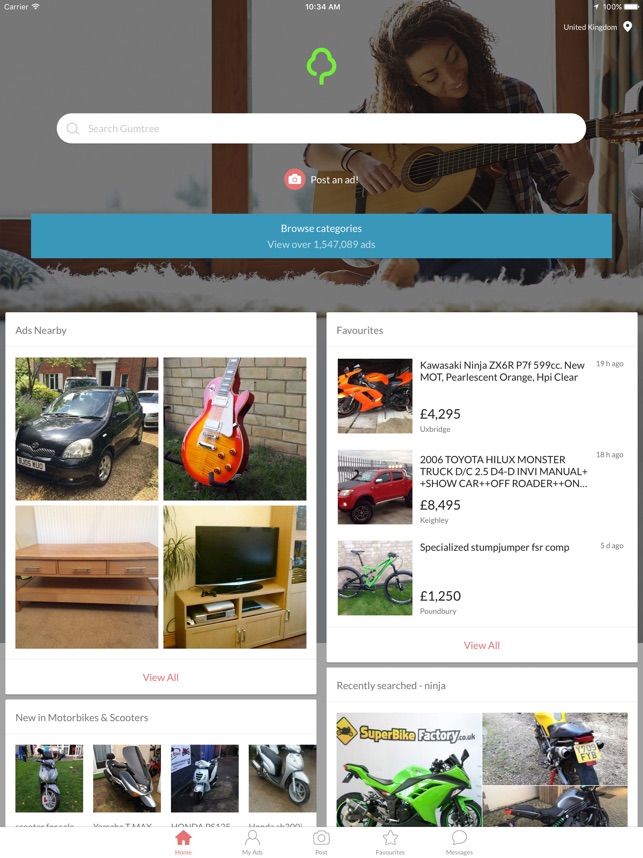This image is a detailed screenshot from a mobile device, showing a comprehensive view of an online ad marketplace. At the top of the image, the status bar indicates the carrier with full signal bars, the time as 10:34 AM, and a fully charged battery icon. Dominating the upper portion is a partial photograph of a young black woman playing an acoustic guitar on a white fuzzy rug, ensconced in a shadowy gray filter. Central to the top half, there is a green tree-shaped logo above a white search bar.

Beneath the search bar, a prominent red circle with a camera icon invites users to "Post an Ad." Adjacent to this, a blue bar with white text reads "Browse Categories," highlighting the vast volume of over 1,547,089 ads. The screen then divides into two sections: 

- **Left Side: 'Ads Nearby'** with a white background and gray text, showcasing images of a car, a guitar, an entertainment center, and a TV on a stand, with an option to "View All." Below this, under the label "New Motor Bikes and Scooters," additional images are displayed.
  
- **Right Side: 'Favorites'** features pictures of a Kawasaki motorcycle, a Toyota vehicle, and a bicycle. Further down, under "Recently Searched," the word "Ninja" and images of Ninja bikes are observed.

At the very bottom of the screen, a navigation bar spans from left to right, featuring icons and text for Home (a red house), My Ads (a user silhouette), Post (a camera), Favorites (a star), and Messages (a speech bubble). The colors and elements blend white, blue, black, and gray, with touches of orange, green, red, and purple scattered throughout, creating a vibrant and organized interface.